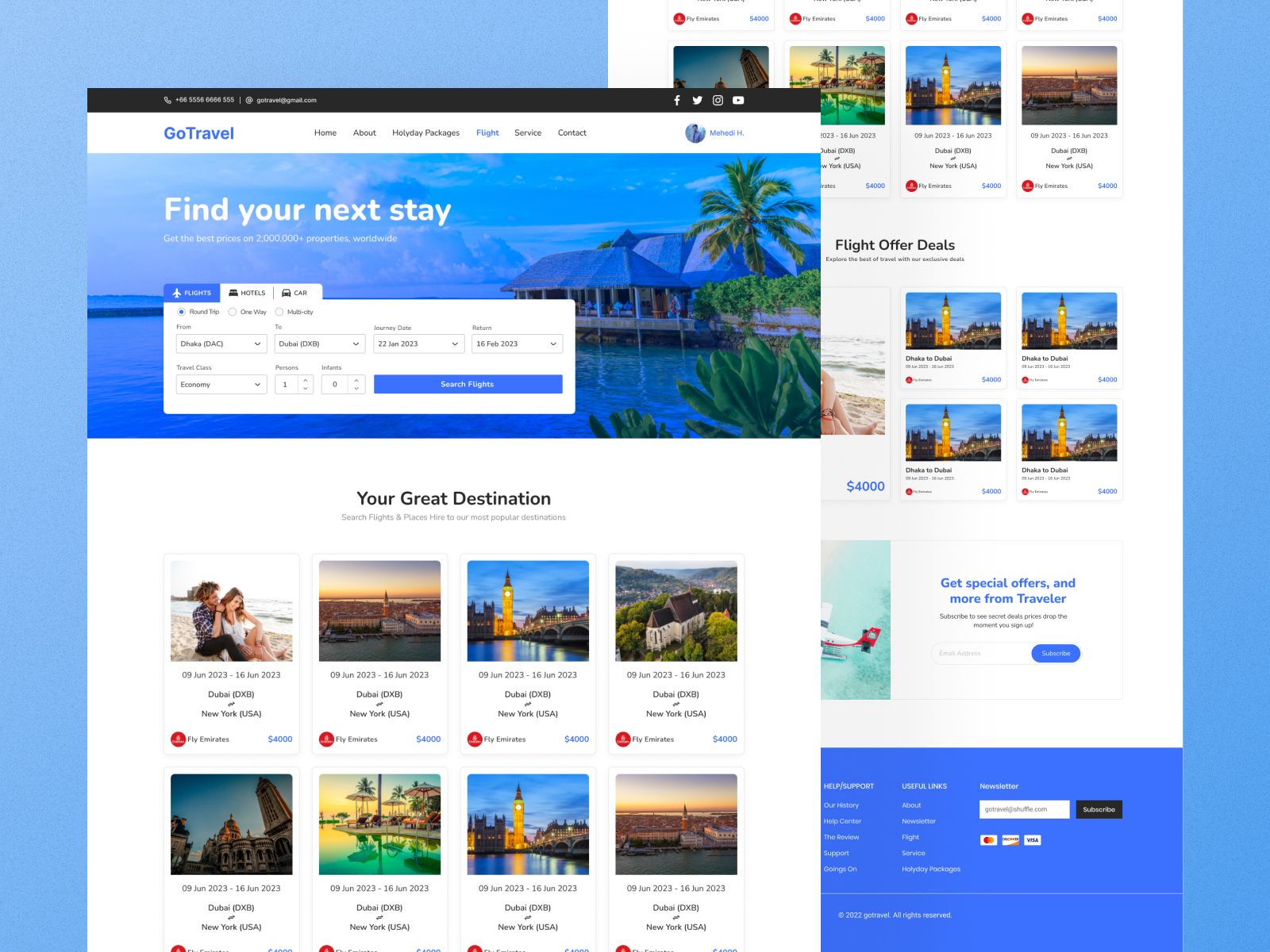The image depicts a travel-themed website with a predominantly light blue background. Dominating the foreground is a web page, positioned slightly to the left. The top section features a black banner, showcasing logos for Facebook, Twitter, Instagram, and YouTube on the right-hand side.

Below this black banner is a narrower white banner on the left, displaying the text "Go Travel" in blue. Adjacent to this, there are navigational menus in black text and a small circular area on the right featuring what appears to be a profile picture and name.

The main section of the page prominently displays a picturesque view of an oceanfront scene including a bungalow and palm trees. Below this image, the text reads "Find Your Next Stay," accompanied by a search bar for entering travel preferences. Further down, a section titled "Your Great Destination" presents eight clickable options, arranged in two rows of four, each depicting small images and possibly price information.

In the background, partially obscured by the main page, is another page that includes additional travel photos, along with text promoting flight deals and special offers labeled "Get Special Offers and More from Traveler."